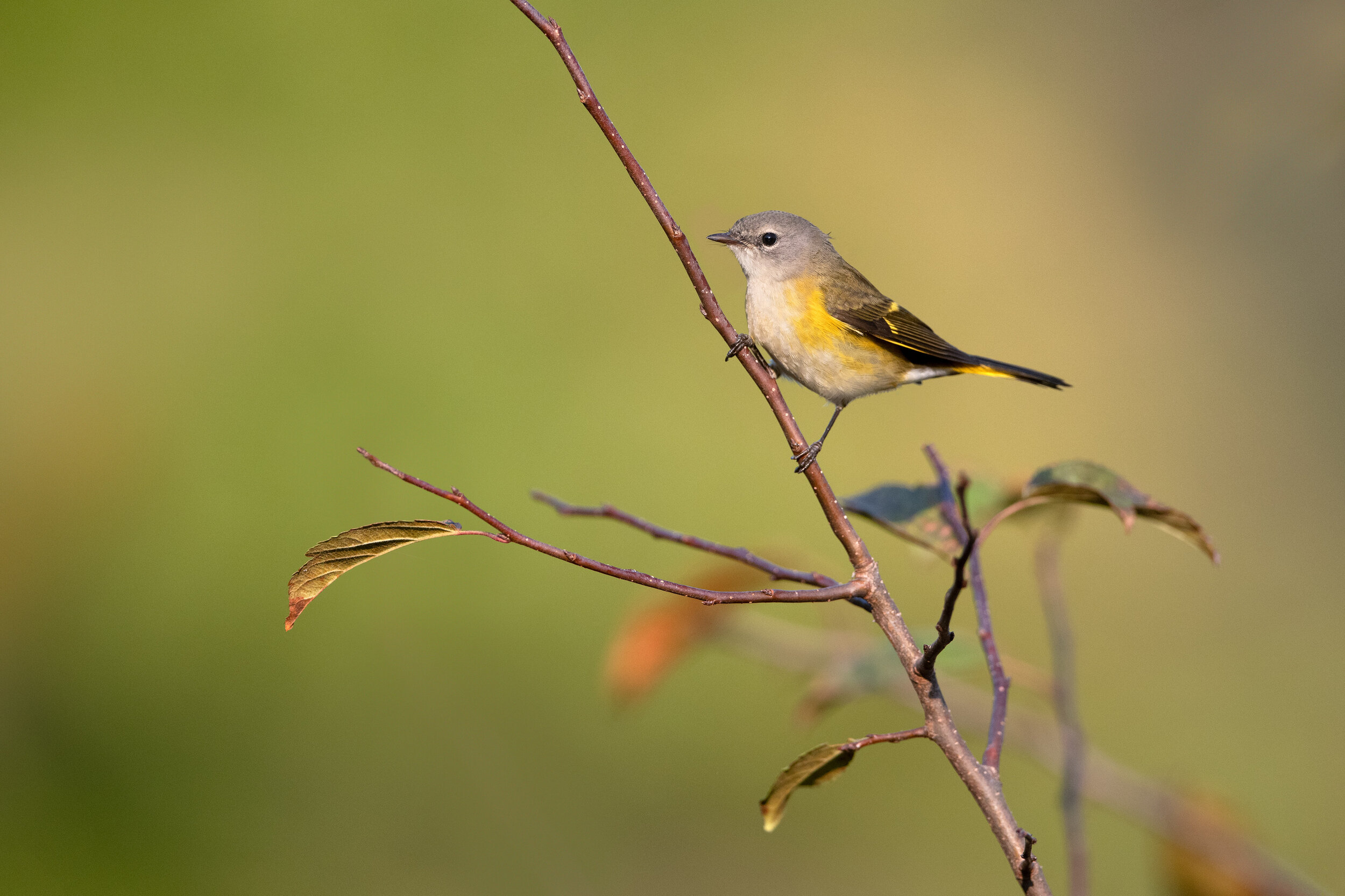In this detailed photograph taken in a natural setting, a small bird, which closely resembles a finch, perches gracefully on a thin, brown branch that extends vertically from the bottom to the top of the image. The bird’s plumage is a beautiful mix of colors: it has a gray head and beak, white around the eyes, a white chest, yellow sides, and striking gray and black wings adorned with hints of yellow. The wings also have a touch of brown, and its tail feathers are black with yellow underneath. The bird’s slender, gray legs grip the branch effortlessly, as it faces the left side of the frame.

The background of the image is a soft, blurred haze of greens with browns and yellows, making it impossible to distinguish any specific elements, thus drawing all the attention to the bird and its perch. One can discern another out-of-focus branch with some leaves behind the bird. The primary branch on which the bird stands also has two leaves on the left side, with additional small branches extending to the right and back. This detailed and focused depiction of the bird on its perch against the indistinct background creates a serene, picturesque snapshot of nature.